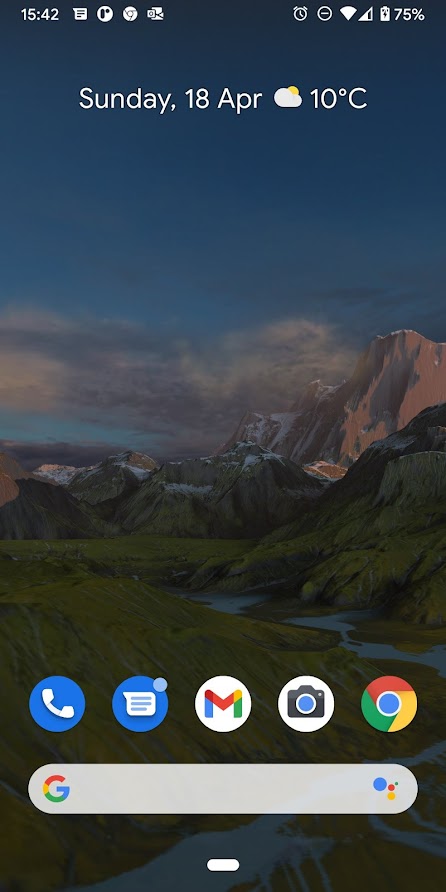This image appears to be a scenic photograph captured using the front camera of a cell phone. Dominating the view is a serene and picturesque landscape. The background features a brilliant blue sky that gradually transitions into a lighter shade as it approaches the horizon. Wispy clusters of low-lying clouds, predominantly white with hints of gray, are scattered across the sky, adding texture to the expanse.

To the right side of the image, a majestic range of snow-capped mountains stands tall, their peaks enveloped in a blanket of white. Contrastingly, the terrain to the left showcases lush green mountains. Interspersed between the mountains, there is a tall, verdant hill set against the snowy backdrop on the right, while another green hill lies lower and further out in the landscape.

In the foreground, a tranquil blue stream winds its way through the valley, cutting through the greenery and adding a sense of depth and movement to the scene.

Overlaying this picturesque view is the phone's interface. At the top-left corner, the time is displayed as 15:42. Adjacent to the time, on the right, the battery icon indicates a 75% charge. Below them, additional details show the date, Sunday 18th April, accompanied by a weather widget depicting a white cloud with a sun peeking behind it and a temperature of 10 degrees Celsius.

Towards the bottom of the screen, several app icons are visible: a white phone in a blue circle, a white notebook paper icon also in a blue circle, an "M" symbolizing Google Mail, and a black camera icon within a white circle. Beneath these icons, a long search bar is prominently displayed, marked by the Google "G" on the left and a small blue circle on the right.

The overall composition blends the natural beauty of the landscape with the familiarity of a smartphone's interface, creating a striking yet relatable image.